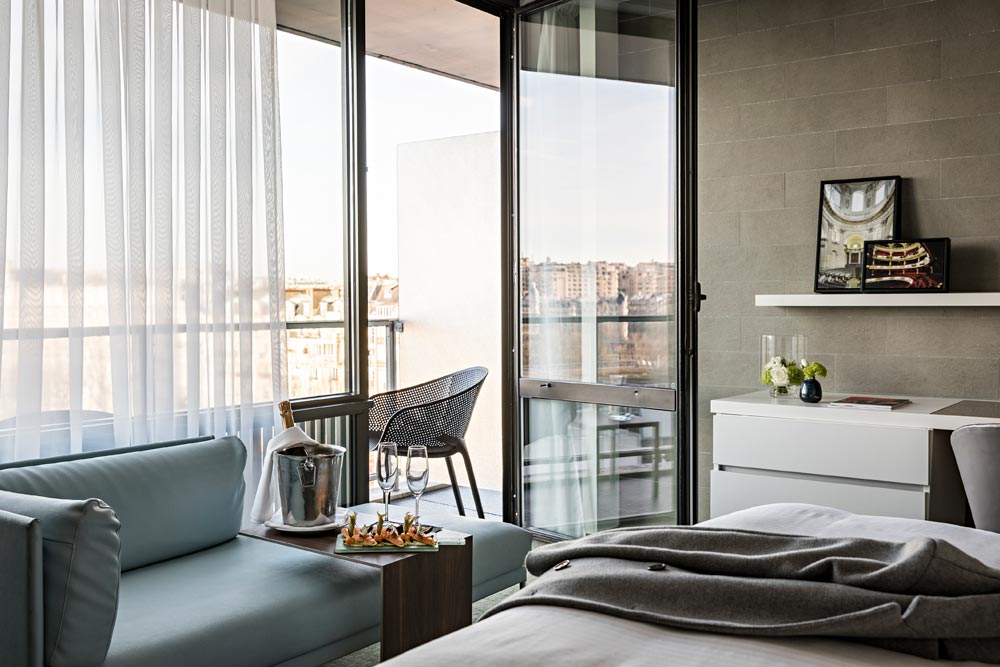This image is a detailed color photograph of a modern, sophisticated hotel bedroom with a balcony, positioned in a landscape layout. On the left-hand side, an open glass door leads to the balcony where there's a black chair and a black railing, allowing a view of the distant cityscape with high-rise buildings. Along the wall of the balcony hangs a thin white drape.

Inside the room, near the balcony door, a light gray couch is complemented by a side table adorned with a stainless steel ice bucket, a bottle of champagne, and two champagne glasses, along with a small tray carrying appetizers. The centrally located bed, dressed in white sheets, features a gray woolen coat casually draped over a gray blanket at its end. In the upper right section of the room, a white desk with plants and a white shelf holding a framed picture stand against a clean, modern gray wall made of what appears to be concrete blocks. Despite the industrial material, the room exudes a sleek and inviting ambiance, making it an elegant retreat within the bustling city.